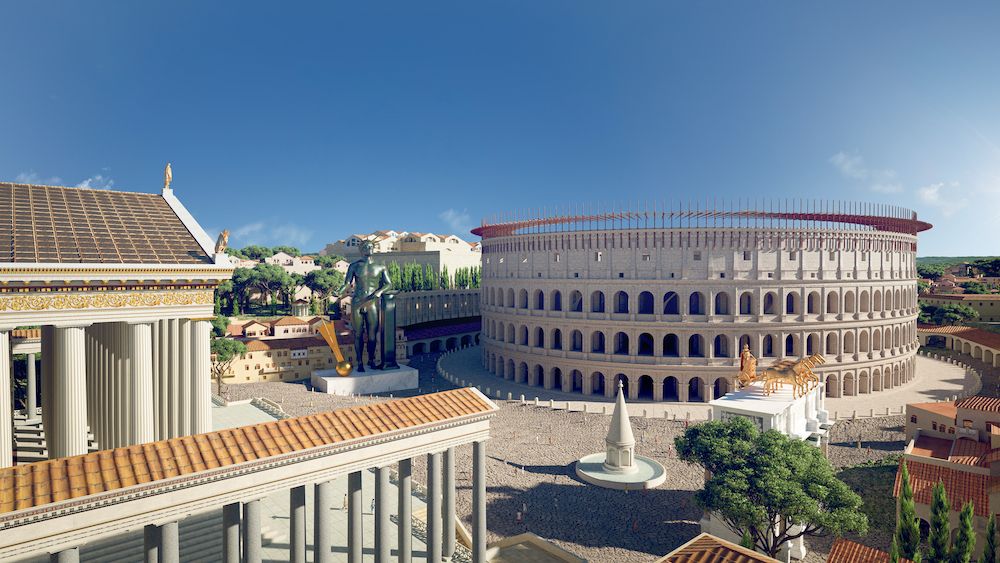In the foreground, a grand coliseum-like structure dominates the right side of this photograph. This circular, white edifice, reminiscent of ancient Roman architecture, features three tiers of arches that encircle the building, each level adorned with numerous window-like openings. The setting appears to be under construction or amidst some unfinished groundwork, highlighted by the surrounding concrete and patches of dirt.

To the left, additional buildings rise, their columnar forms topped with triangular roofs. These structures, alongside the coliseum, suggest an array of classical architectural influences. A large open area in front of the coliseum, potentially a gathering space, is marked by a prominent statue or monument reminiscent of a spear. 

The scene is bathed in bright daylight, with a clear blue sky punctuated by just a few patchy clouds, enhancing the vibrant color palette of off-white, tan, brown, green, and various shades of blue and beige. The photo appears to have been taken from an elevated vantage point, offering a comprehensive view of this architectural tableau. Surrounding the scene, tall buildings with orange-tiled roofs and lush trees frame the historical ambiance, suggesting a foreign locale dedicated to preserving or celebrating ancient styles. There are even flags adorning the coliseum, contributing to the historical aura of the setting.